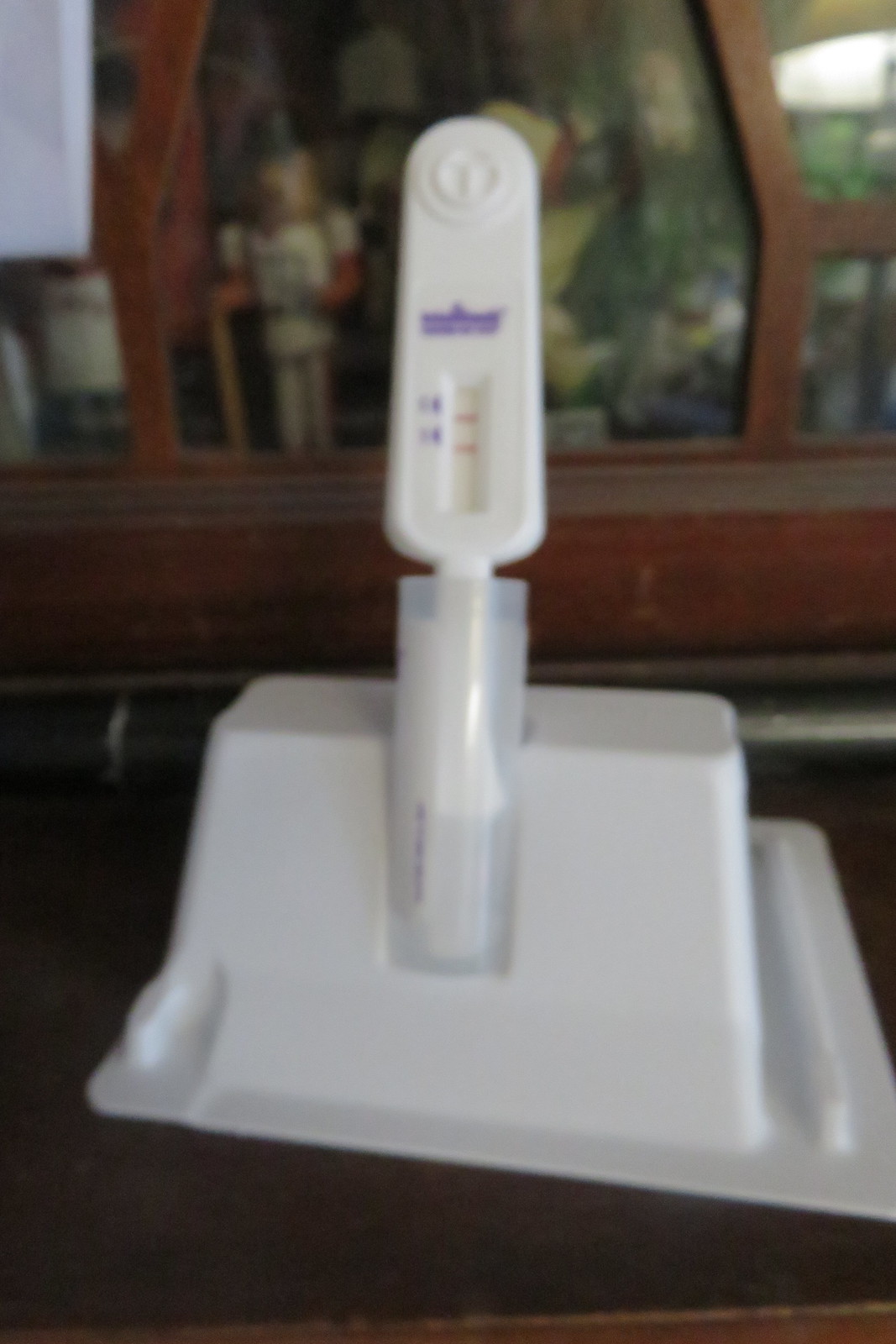The image showcases a close-up view of a home-based medical test kit. Central to the composition is a rectangular, white, flat plastic tube, inserted into a transparent specimen bottle. The specimen bottle is secured within a plastic holder. The design suggests functionality akin to that of a home pregnancy test kit. Prominently displayed at the front of the device are a series of numbers and two red indicator lines. The test kit is placed on a rustic brown wooden surface. In the background, a wooden frame adorned with photographs adds a homey touch to the setting.